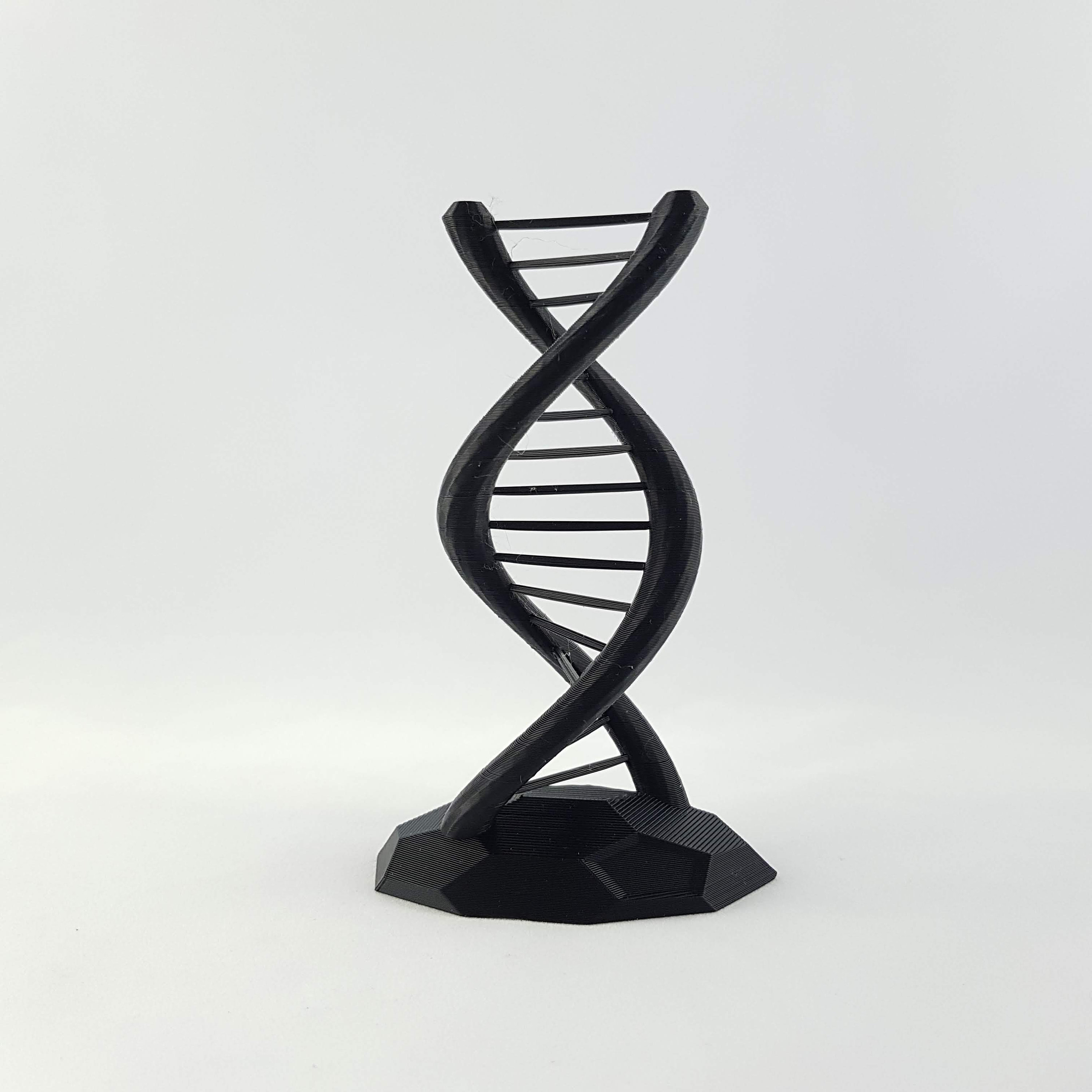This image features a black sculpture of a DNA helix set against a white background and placed on a white surface. The helical structure, easily recognizable as a model of a DNA strand, includes two large spiraling sides intertwined by rods that represent the amino acids—adenine (A), guanine (G), cytosine (C), and thymine (T). The sculpture, viewable from a top-down angle showing the strands spinning counterclockwise, sits singularly in the image with no other objects surrounding it. The entire model is mounted on a sturdy black base, and the photograph is in black and white, highlighting the intricate, twisting structure of the DNA helix.